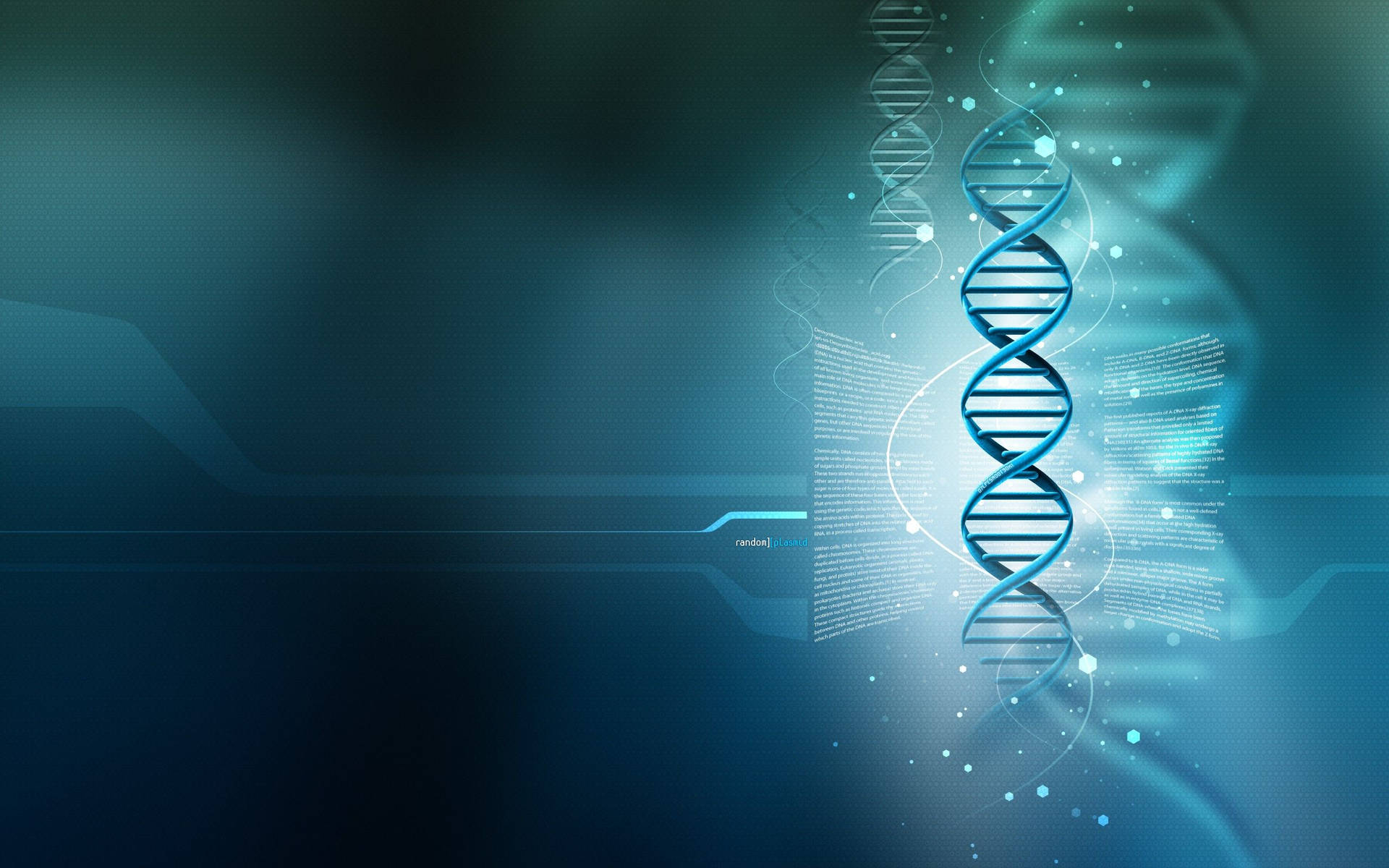This image, predominantly featuring various shades of blue—from aqua to dark midnight blue—depicts a highly detailed, computer-generated representation of a DNA strand. The DNA helix, which appears in a lightish blue, stands out centrally amidst darker blue backgrounds and horizontal lines of varying thicknesses. These lines lead towards clusters of small, faint, and mostly illegible white text, with three paragraphs situated to the left and four to the right. The text is dwarfed by the central, interlocking blue swirls of the DNA strand, which are accentuated by surrounding strings and dots of light as well as a distinct white line of light visible behind the helix. Additionally, there's a ghost image of a shorter DNA chain to the upper left, appearing more faded. Words such as "Random Plasmid" are partially legible, with "Random" in white and "Plasmid" in a dark blue hue, situated towards the bottom left side of the image. The entire composition creates a vivid, dynamic visualization of genetic material amidst an abstracted, science-themed background.